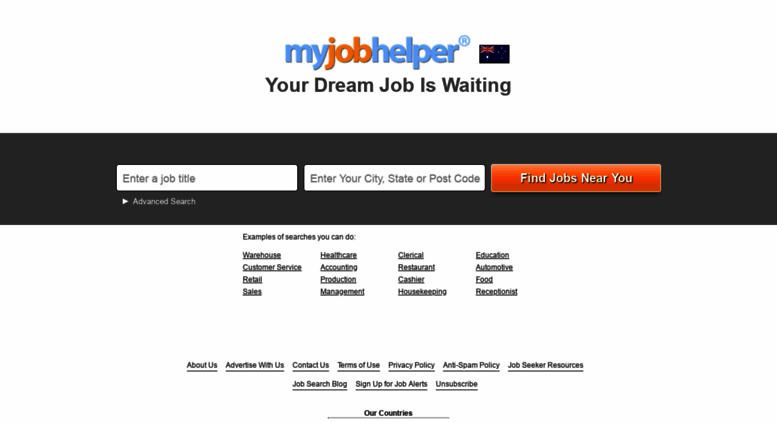The image is a horizontally rectangular frame with a primarily white background. At the top center of the frame, the text "My Job Helper" is prominently displayed, with "My" and "Helper" in light blue and "Job" in orange. Below this title, in dark gray text, it reads, "Your Dream Job is Waiting."

Directly underneath this phrase is a dark gray horizontal banner that extends the width of the frame. Within this banner are two adjacent white input fields. The first field on the left is labeled "Enter a Job Title," and the one to its right is labeled "Enter Your City, State, or Postcode." Further to the right is an orange button with the text "Find Jobs Near You" in white.

Beneath the banner, the white background continues, featuring the title "Example of Searches You Can Do" with each example listed as an underlined, clickable link. The job categories listed include Warehouse, Customer Service, Retail, Sales, Healthcare, Accounting, Production, Management, Clerical, Restaurant, Cashier, Housekeeping, Education, Automotive, Food, and Receptionist.

At the bottom of the image, multiple page option links are displayed: About Us, Advertise With Us, Contact Us, Terms of Use, Privacy Policy, Anti-Spam Policy, Job Seeker Resources, Job Search Blog, Sign Up for Job Alerts, and Unsubscribe. Centered at the very bottom of the frame is the text "Our Countries."